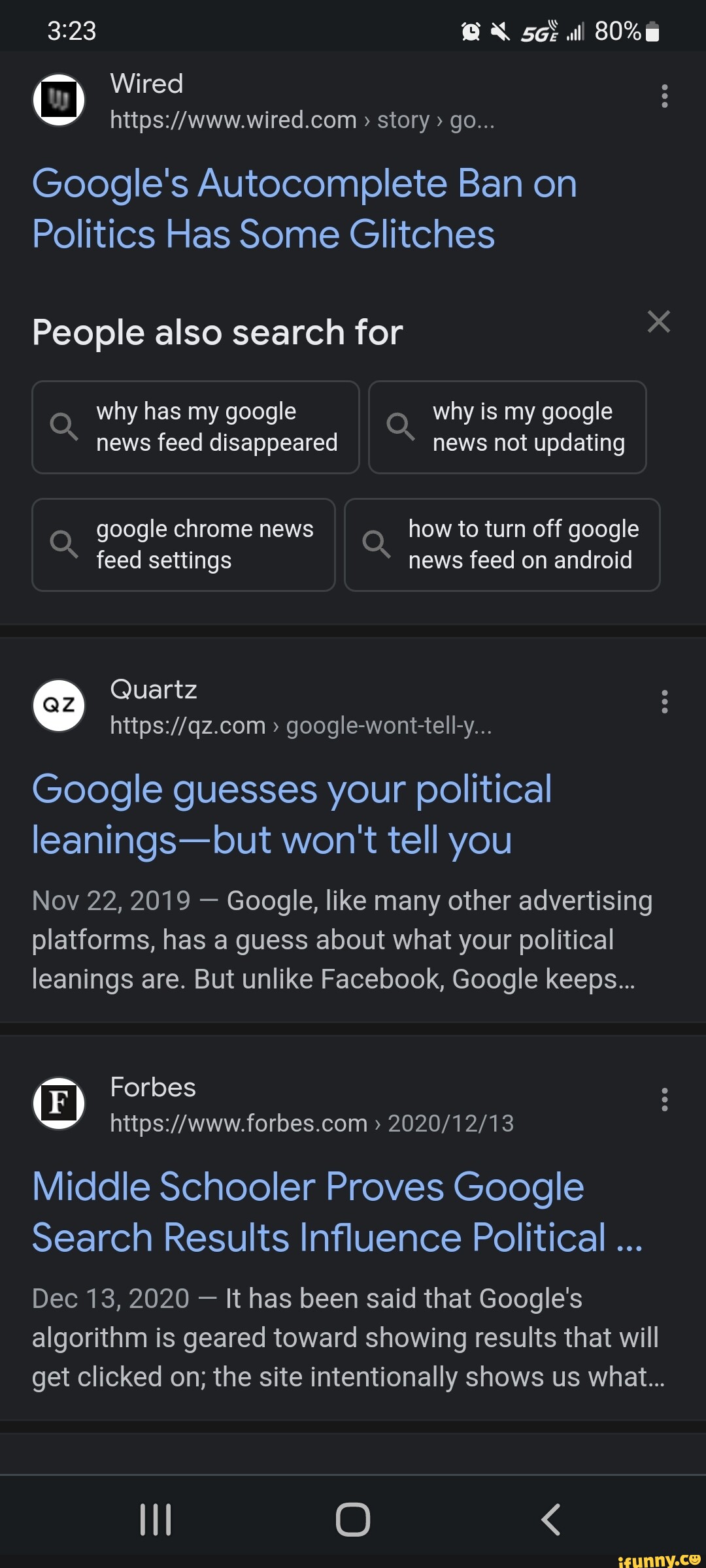The image is a screenshot of a Google search results page displayed on a device with a black background. At the top of the screenshot, the status bar shows the time as 3:23 and includes standard icons for a phone's status indicators.

The webpage being viewed is from Wired, as indicated by the URL "www.wired.com" visible in the address bar. The main search result is highlighted in blue and reads, "Google's auto-complete ban on politics has some glitches." Beneath this title, in white text, it says "people also search for," followed by four suggested queries:
1. "Why has my Google News feed disappeared?"
2. "Why is my Google News not updating?"
3. "Google Chrome News feed settings"
4. "How to turn off Google News feeds on Android"

Further down, two articles from different sources are listed as additional search results. The first article is from Quartz, denoted by the "QZ" icon inside a white circle. The title of this article is "Google guesses your political leanings but won’t tell you," with a brief excerpt following the title. The second article is from Forbes, marked by a white "F" inside a black box. The title reads, "Middle schooler proves Google search results influence political..." with an excerpt also provided.

These elements combine to offer a detailed snapshot of the search results for a query related to Google's handling of political content in its auto-complete feature.